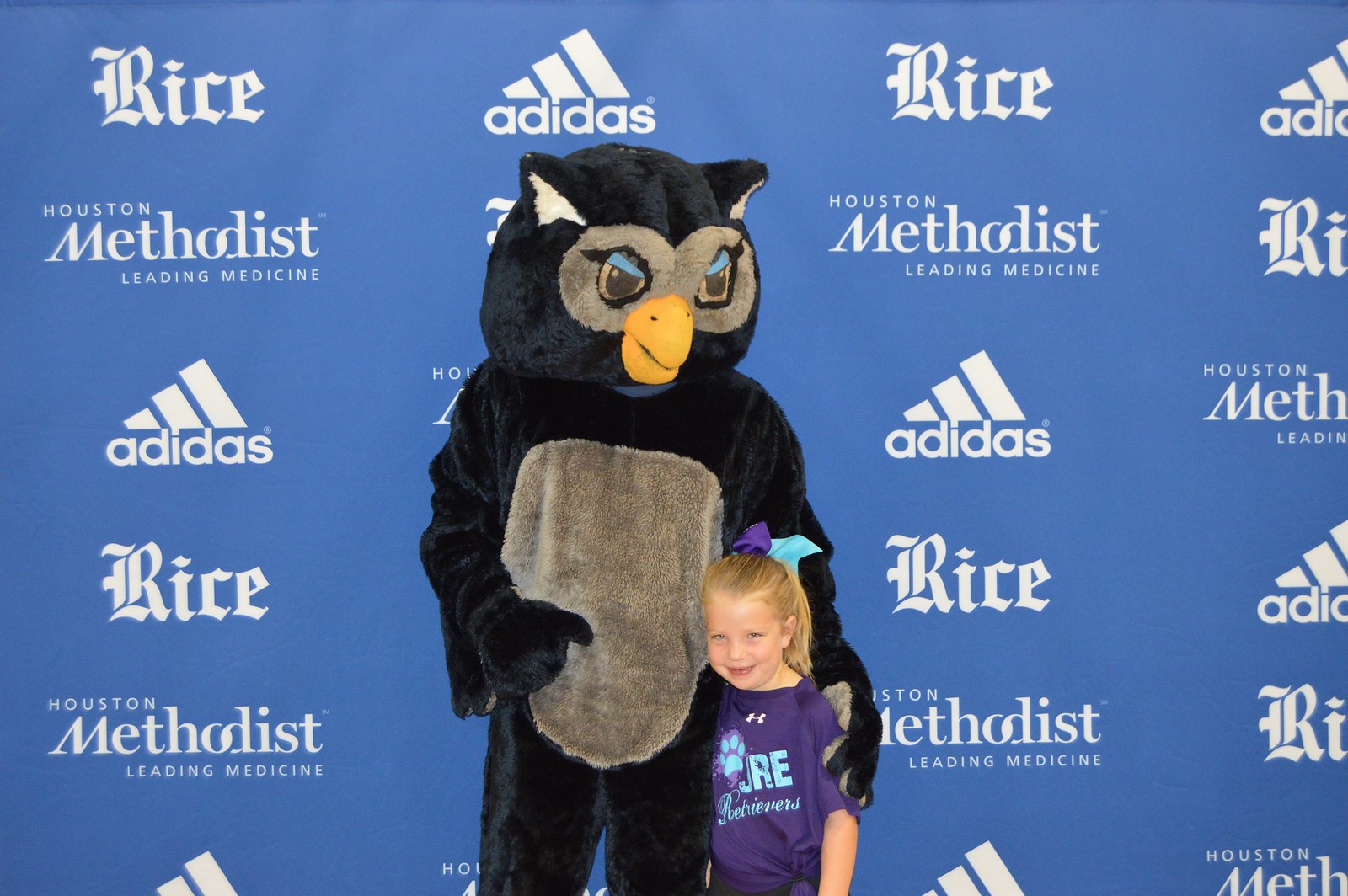In this image, a mascot and a young girl are standing in front of a large blue banner adorned with repeating sponsor logos. The banner predominantly features the names "Rice," "Adidas," and "Houston Methodist Leading Medicine" in white text against the blue backdrop, arranged in alternating lines.

The mascot is an owl characterized by a black head, white ears, gray eye markings, dark eyes, an orange beak, a black body, and a gray stomach. It has a friendly demeanor and has its arm around the young girl. The girl, estimated to be around five or six years old, has blonde hair adorned with a purple and turquoise bow. She is wearing a purple t-shirt with turquoise lettering on the front. The duo stands out vibrantly against the professional backdrop, creating a charming and engaging scene.